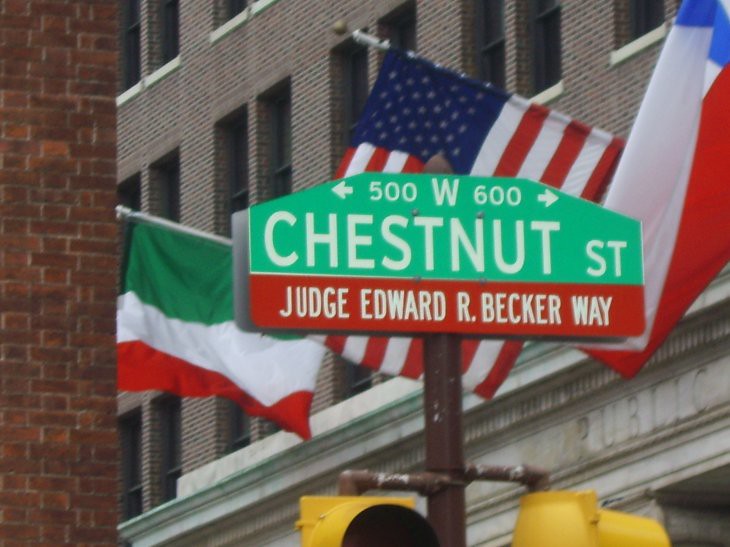This color photograph captures an upward view of the upper part of a gray stone building, likely its second or third floor. Visible in this shot are several windows, partially obscured by overhanging flags situated above the building's entryway. Prominently in the center is the U.S. flag with its iconic stars and stripes. On the right, although only partially visible, is a flag featuring large white and red stripes. The third flag, composed of three horizontal stripes in emerald green, white, and red, is also not fully identifiable.

Foregrounding the scene is a prominent street sign that obstructs a clear view of the flags. The top part of the sign, colored green with white letters, reads "Chestnut Street," with "ST" as the abbreviation for "Street." Displayed above this text is "500," accompanied by a left-pointing arrow, while "W" and "600" with a right-pointing arrow are listed below.

Beneath the green portion, a red strip displays "Judge Edward R. Becker Way" in bold white letters. The detailed signage provides a visual reference for the location within the urban landscape.